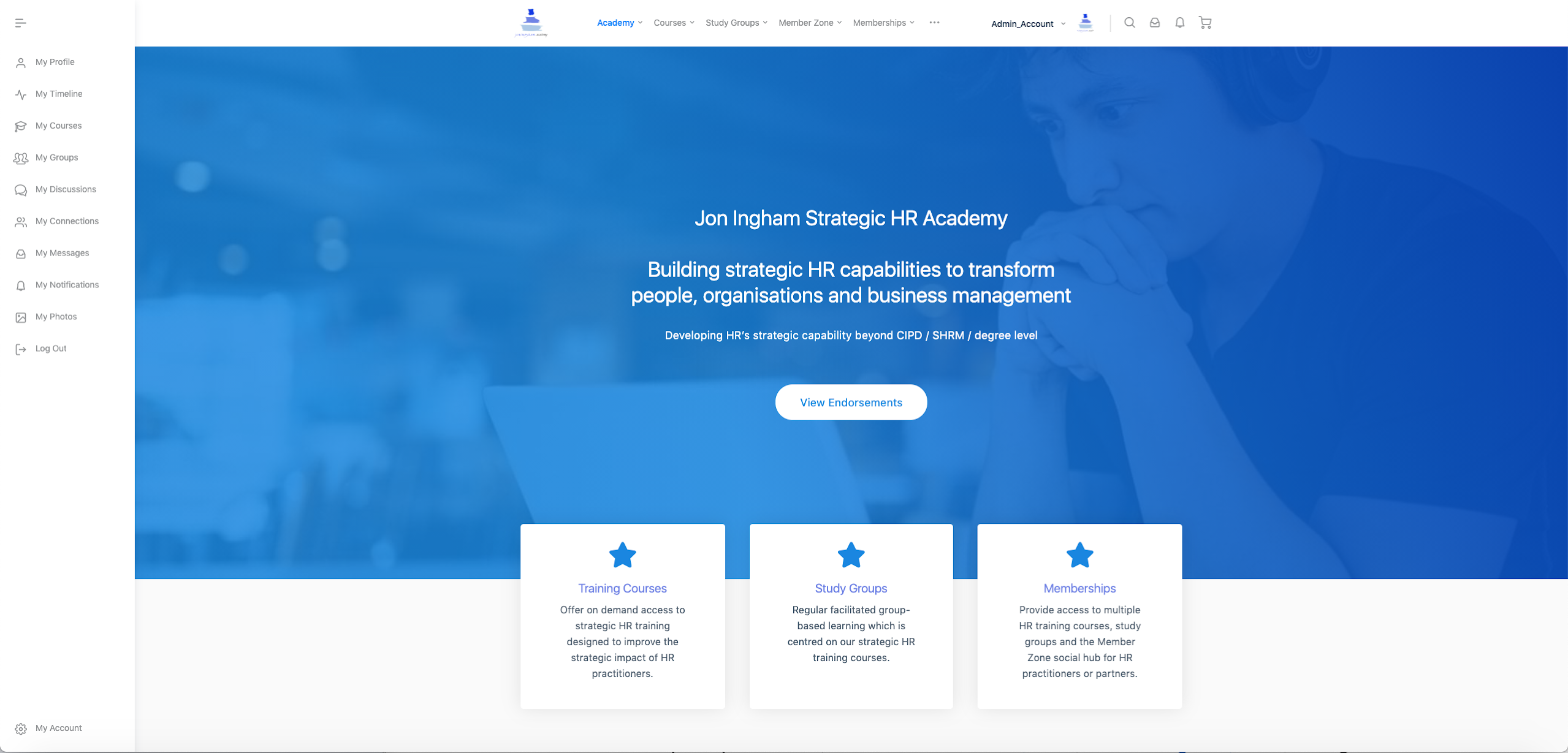The image features a prominent blue rectangle in the center, which contains the text: "John Ingram Strategic HR Academy - Building Strategic HR Capabilities to Transform People, Organizations, and Business Management." Beneath this rectangle, there is a smaller white, oval-shaped circle featuring the text "View…" (the remaining text is unclear).

Below the blue rectangle are three white squares, each topped with a star. These squares contain additional text, although the font is very small and difficult to decipher.

On the left side of the blue rectangle, vertical text appears in a column, accompanied by emblems corresponding to each set of words. However, both the words and the emblems are too small to be read clearly.